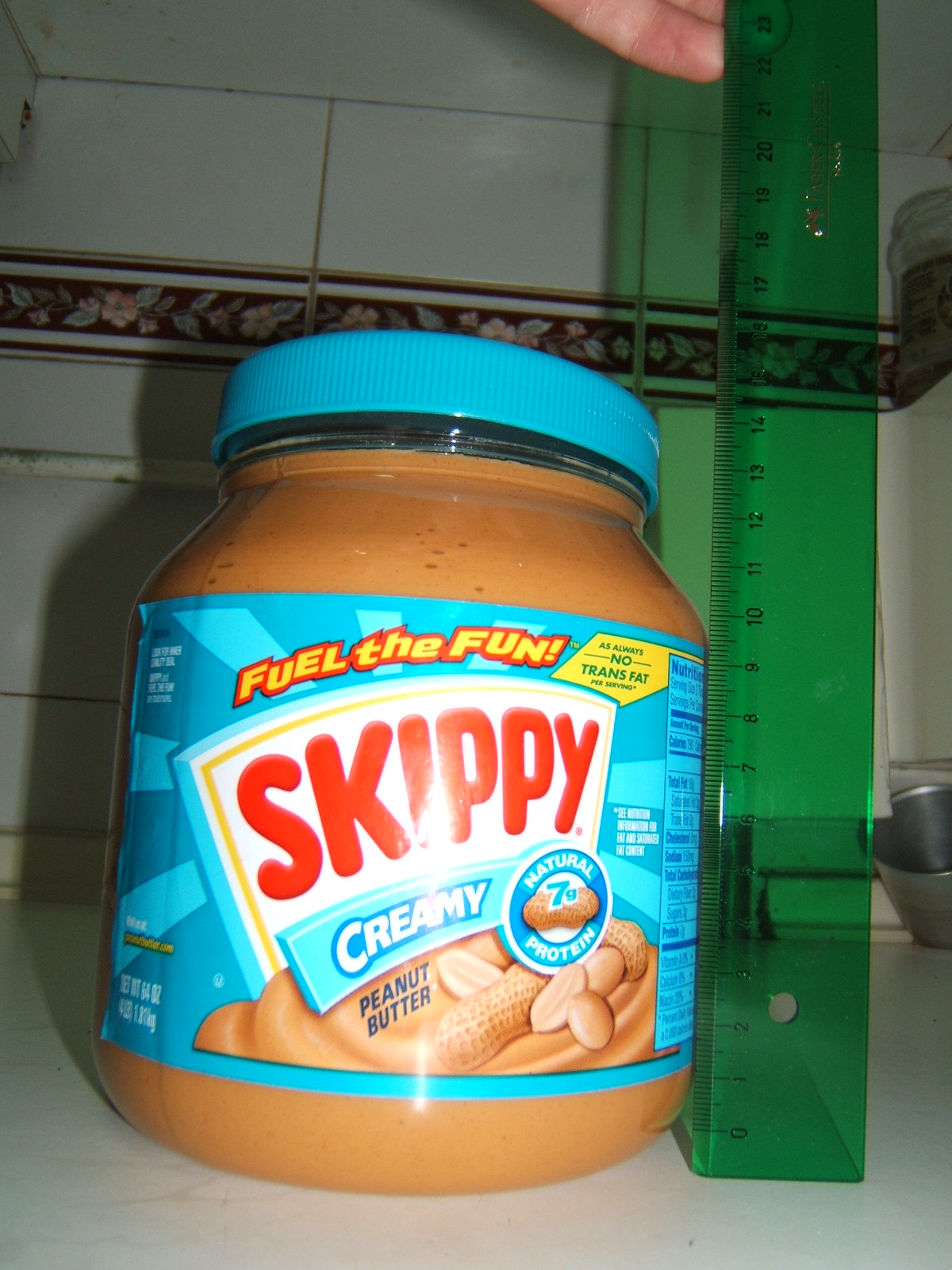A vibrant image showcasing a container of Skippy Creamy Peanut Butter. The label prominently features cheerful yellow text with a red outline, declaring "Feel the Fun" and highlighting that the product contains "No Trans Fat." The container itself bears a blue label and is sealed with a light blue lid. Beside the peanut butter jar, a green ruler is held upright by a person, providing a sense of scale. The background contrasts with a simple white hue, ensuring the focus remains on the playful and enticing Skippy packaging.